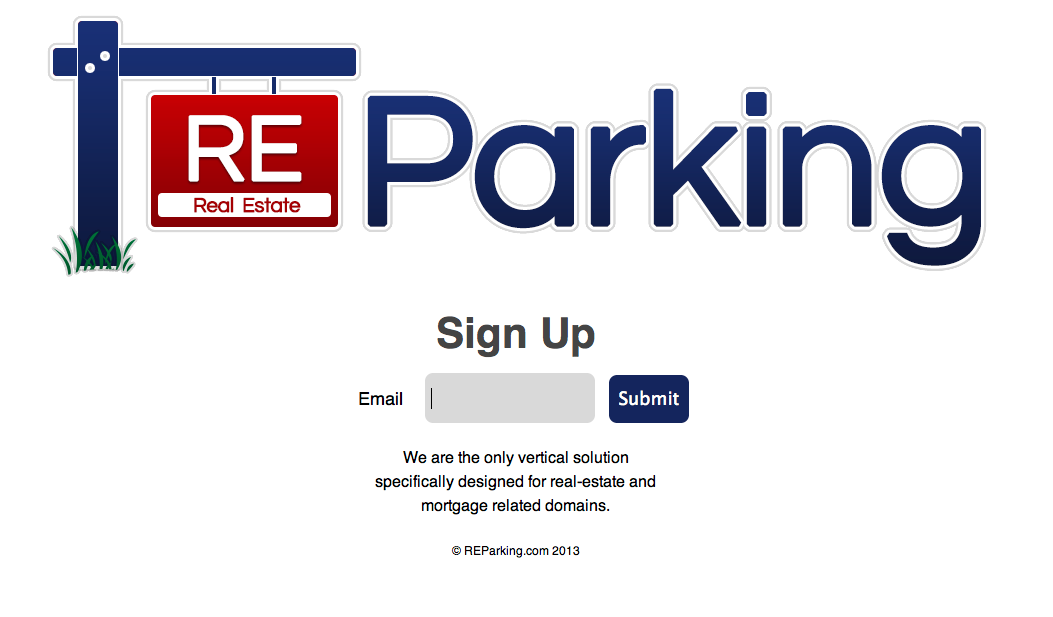This illustration features a few sprigs of grass situated next to a wooden post with an attached arm. The post and sign are artistically drawn rather than photographed. The sign is red and prominently displays the text "RE Real Estate" in large, navy blue letters. Below this, an invitation to "sign up" is written, accompanied by a field labeled "email" for entering an email address. Adjacent to this field is a navy blue button with white text reading "submit." The bottom of the sign includes the tagline, "We are the only vertical solution specifically designed for real estate and mortgage-related domains," followed by the URL "reparking.com2013." The overall scene maintains a clean and minimalistic design, focusing on the informational sign and subtle natural elements.